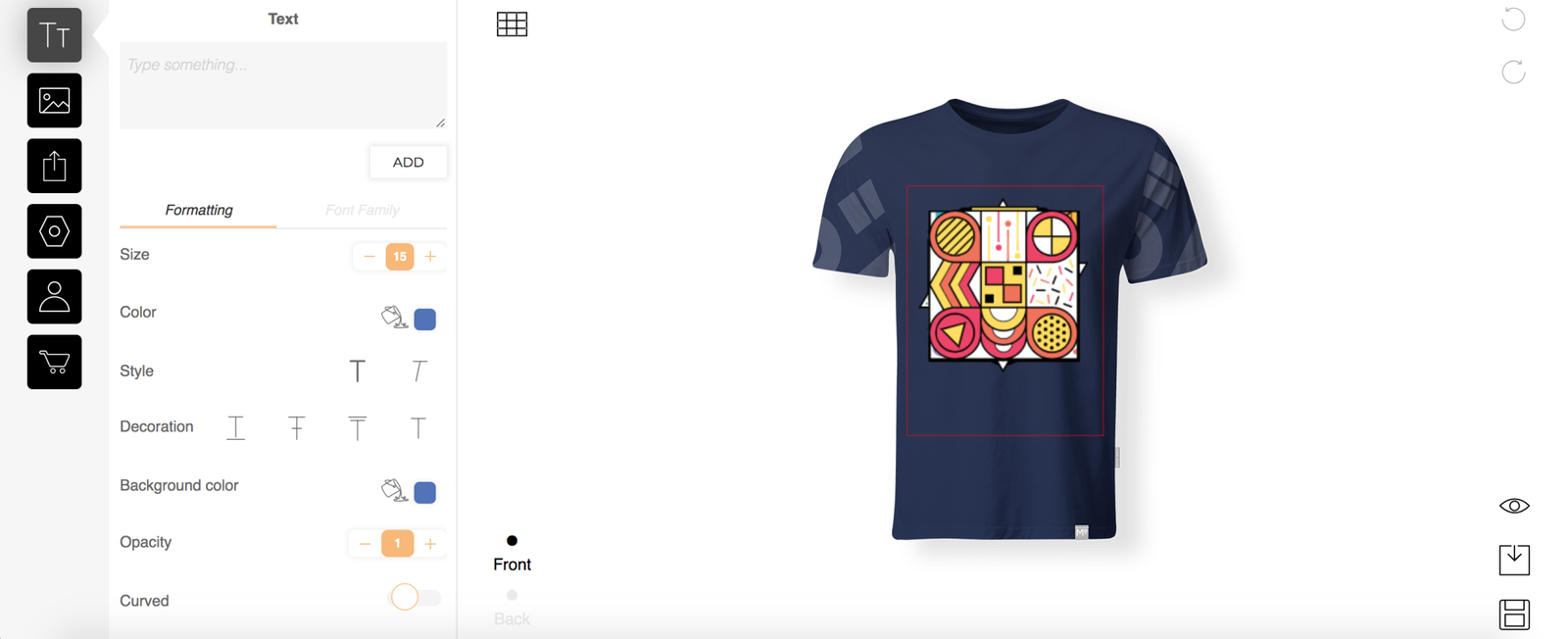The image depicts a user shopping for a shirt on a website. On the left side of the screen, there is a vertical light gray sidebar containing several icons: a photo icon, download icon, settings icon, profile icon, and a cart icon, all displayed in black against white squares.

In the main section of the screen, the interface features a white background. Approximately two inches from the left sidebar, there is black text and a light blue rectangle prompting the user to "Type something". To the right of this prompt is a white tab with the word "ADD" in all capital letters, written in black. Below this input area, the word "Formatting" is displayed in black, underlined with red or yellow. Beneath it, various formatting options are listed in gray: "Font family," "Size," "Color," "Style," "Decoration," "Background color," "Opacity," and "Curved." Adjacent to these labels are corresponding selection options.

On the right side of the screen is a preview section featuring the shirt. In the upper left corner of this section, there is a 3x3 grid of squares. Centered in this area is a dark blue, almost purplish shirt with gray sleeves. A square design with red and yellow patterns is prominently displayed on the front of the shirt. Below this, a black dot is marked with the word "Front" in black text. In the bottom right corner, additional icons—an eyeball icon, a download icon, and a disc icon—are all rendered in black.